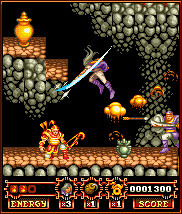This is a pixelated screenshot from a retro 8-bit or 16-bit style video game, depicting a dynamic scene with vibrant, stylized elements. The floor appears to be made up of bubbles or a reddish stone pattern, enhancing the whimsical yet gritty atmosphere. A large, muscular character clad in yellow and red armor kneels with a bow and quiver of arrows. Above this character, another figure is leaping downward while brandishing a weapon, likely a knife-head or a bow, creating an intense action-packed moment. To the left of the scene, floating steps lead to a yellow or golden urn resting on the top step, adding to the mystical environment of stylized trees and explosions. Meanwhile, another warrior in yellow and purple armor, wielding a bloody sword and shield, charges into the frame from the right. At the bottom of the screen, detailed gaming information displays the players' scores and energy levels, alongside some sort of green icon, completing the intricate and chaotic tableau.